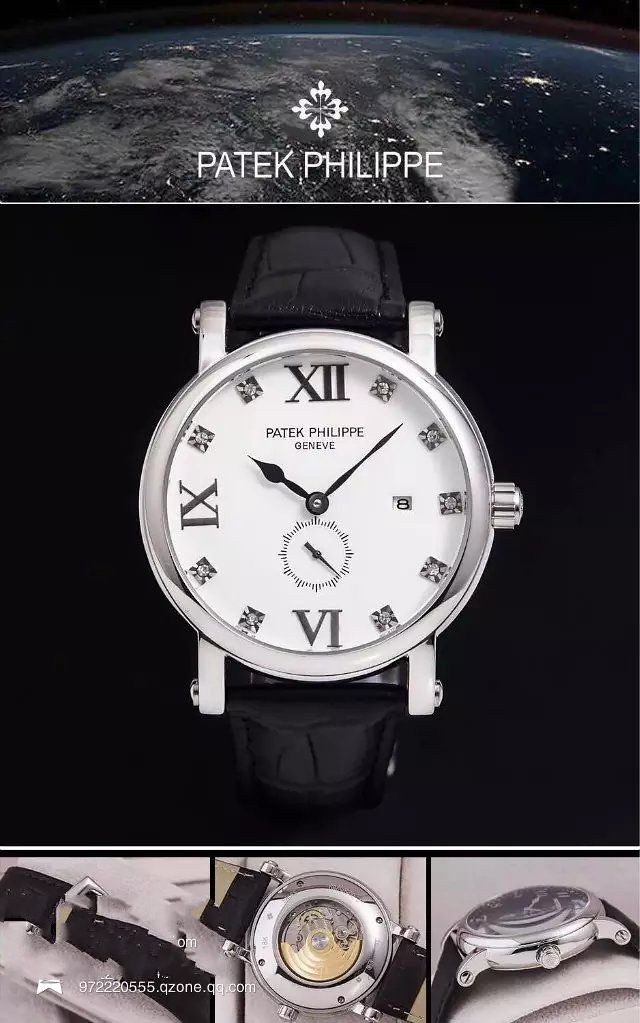The advertisement is a large rectangular poster showcasing a Patek Philippe watch through three distinct images. 

At the top, a rectangular image captures the curvature of the Earth at night, with a black background highlighting the illuminated city lights scattered across the globe. The iconic Patek Philippe logo is prominently displayed in the center of this celestial scene.

The central and largest image dominates the poster, featuring a close-up of a Patek Philippe watch against a stark black backdrop. The watch boasts an elegant white face adorned with diamonds around the circumference, except at the 6, 9, and 12 o'clock positions. It has a sophisticated black leather band. The main watch face reads "1008" and includes a smaller sub-dial seamlessly integrated at the bottom, bordered by delicate lines. A tiny date window is perfectly positioned adjacent to the 3 o'clock area, adding a touch of functional elegance.

At the bottom, a horizontal rectangular strip showcases various detailed images of the Patek Philippe watch or multiple watches, completing the advertisement with a comprehensive view of their exquisite timepieces.